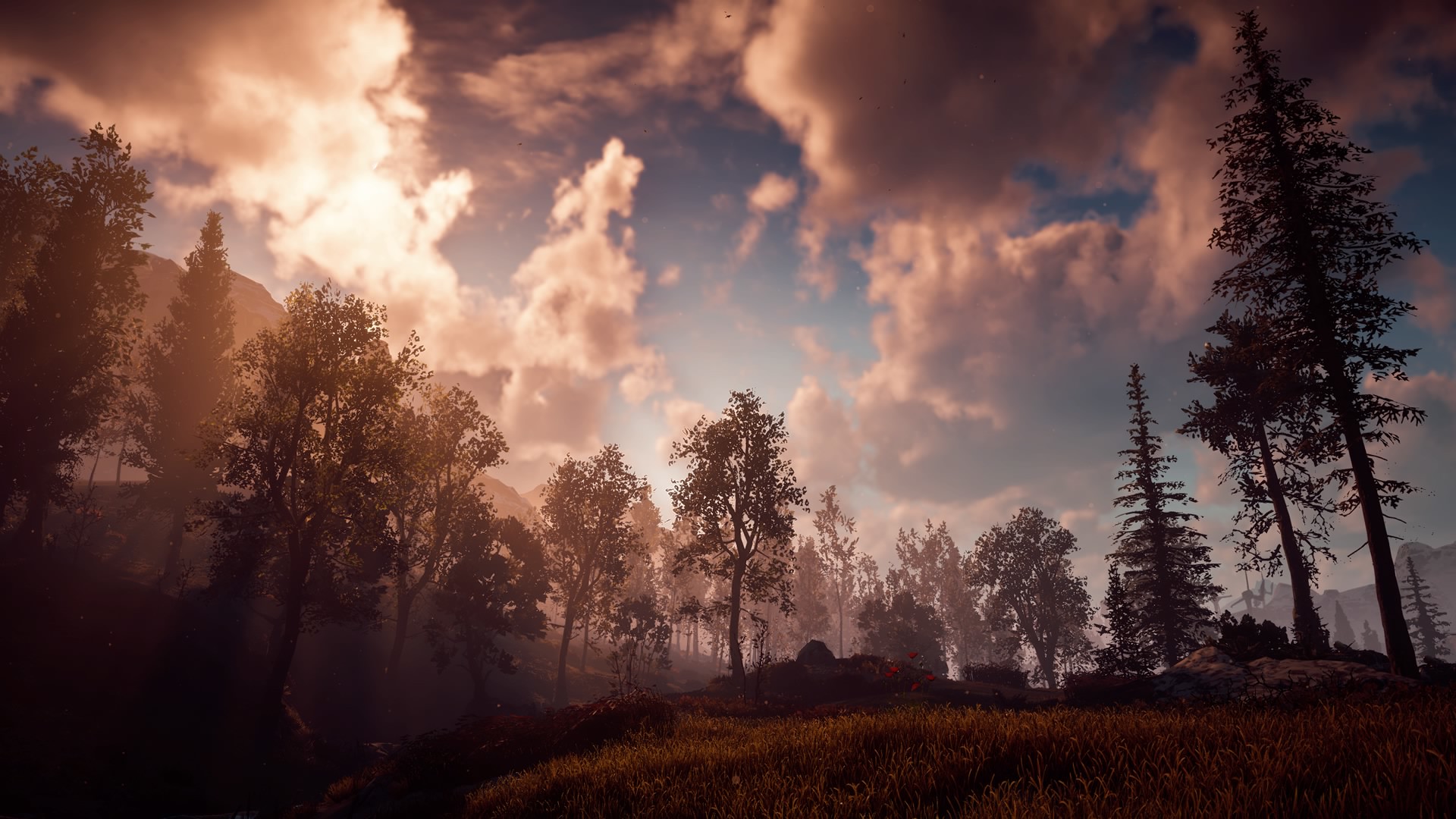This captivating photograph captures a serene forest landscape bathed in the early morning or late evening light. A vibrant blue sky, adorned with well-defined, fluffy, bright white clouds, stretches across the scene. The clouds' undersides are tinged with dark gray shadows, contrasting beautifully with their illuminated upper sections. The forest below is a tapestry of varying tree species, with tall, majestic pine trees standing alongside other deciduous varieties. In the bottom right corner, a gentle hill rises, covered in dark, fluffy grass that catches occasional beams of light. To the far right, distant, blurry mountains peek through the foliage, adding depth and a sense of vastness to the picturesque vista.